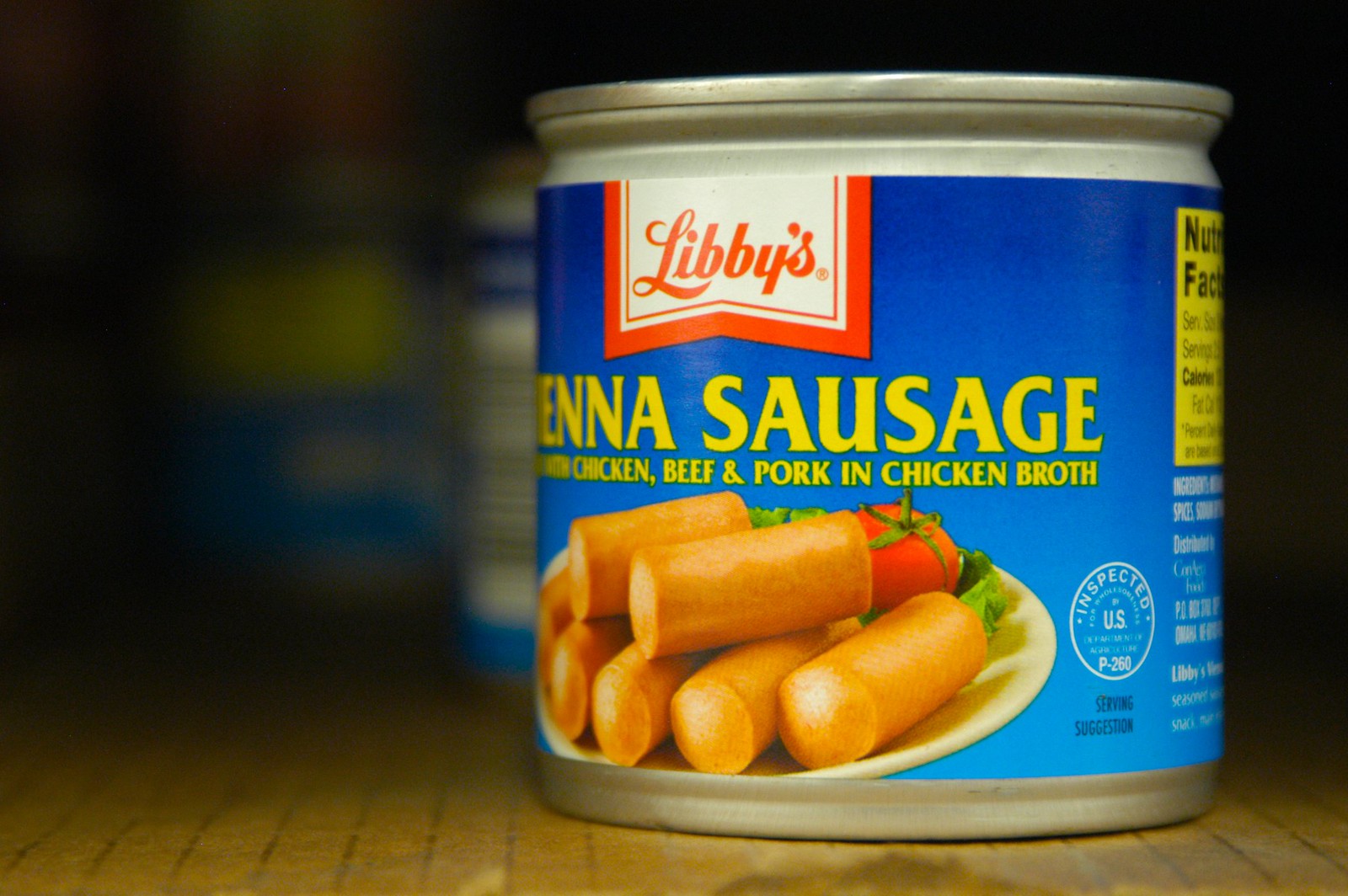The image features a close-up view of a wooden cabinet shelf. The shelf is stocked with various items, primarily canned goods. Dominating the foreground is a sharply focused can of Libby's Vienna Sausage, showcasing its blue label that details the ingredients: chicken, beef, pork, and chicken broth. The nutritional facts are partially visible on the can's right side. In the background, there are two additional items: one is an out-of-focus can, and the other appears to be a blurry jar, possibly containing pickles. The background remains dark, adding contrast and emphasizing the focused can of Vienna Sausages in the forefront.